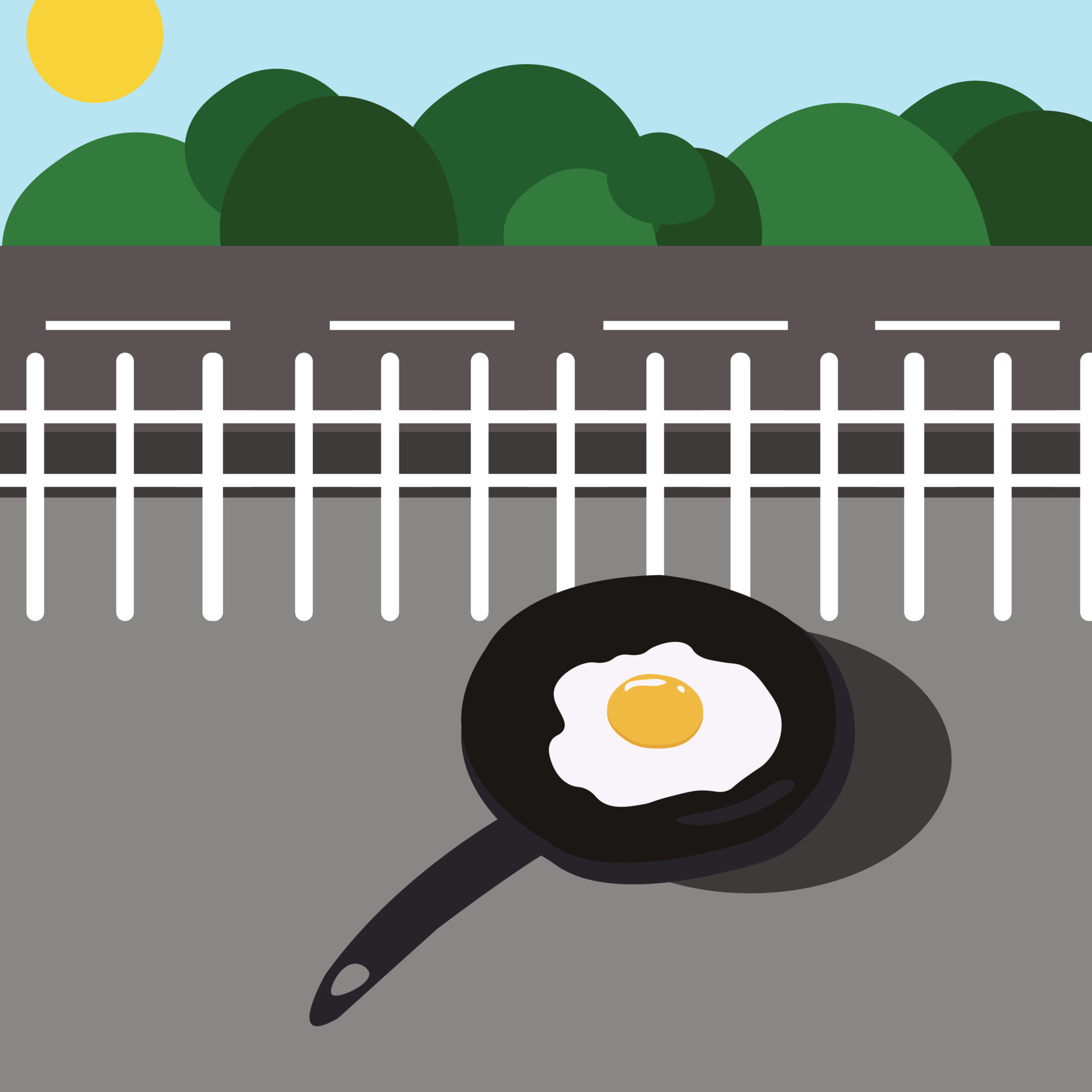The image is a simple yet charming art piece, possibly created digitally or with paint, featuring a vertically rectangular layout with no distinctive border. At the top of the image, a clear blue sky stretches across, unbroken by clouds, with a vibrant yellow sun positioned in the upper left corner. Below this sky, a row of green trees, depicted as varied sizes of green balls and arches, creates a whimsical tree line. A dark gray paved road with white dividing lines runs horizontally below the trees, leading to a white picket fence that spans the middle of the image. In the foreground, a black frying pan with a handle pointing down to the left sits on a gray surface, casting a shadow to its right. Inside the pan, a white egg with a bright yellow yolk appears to be cooking, seemingly heated by the sun above. The overall composition suggests a playful and surreal interpretation of a sunny outdoor scene where the sun appears to be frying the egg in the pan.